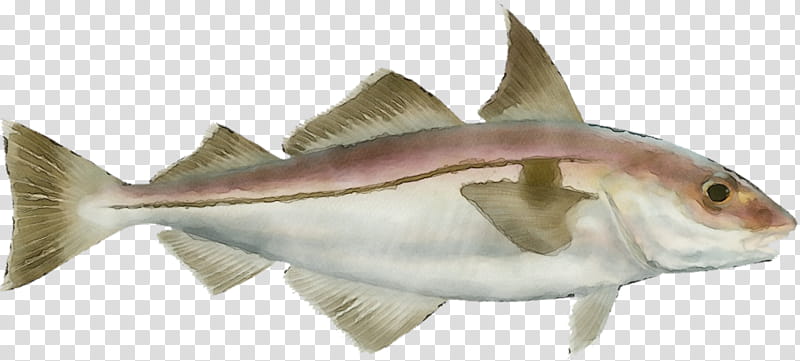The image is a lengthy, horizontally oriented, animated illustration of a fish against a gray and white checkered background, resembling a transparent layer in Photoshop. The fish is positioned facing right. It features a distinct black eye, a white underbelly, and a top that transitions from a pinkish hue to a brownish snout. Its fins—two underneath, three on top, and one on each side—range in color from white to light brown, with those on the undersides being predominantly white and light brown, while the top fins are slightly darker. A subtle greenish line runs through the middle of the fish, and its tail exhibits a brownish-green shade. The illustration gives a three-dimensional impression, as if the fish is viewed from a slight angle below, placed on a board.